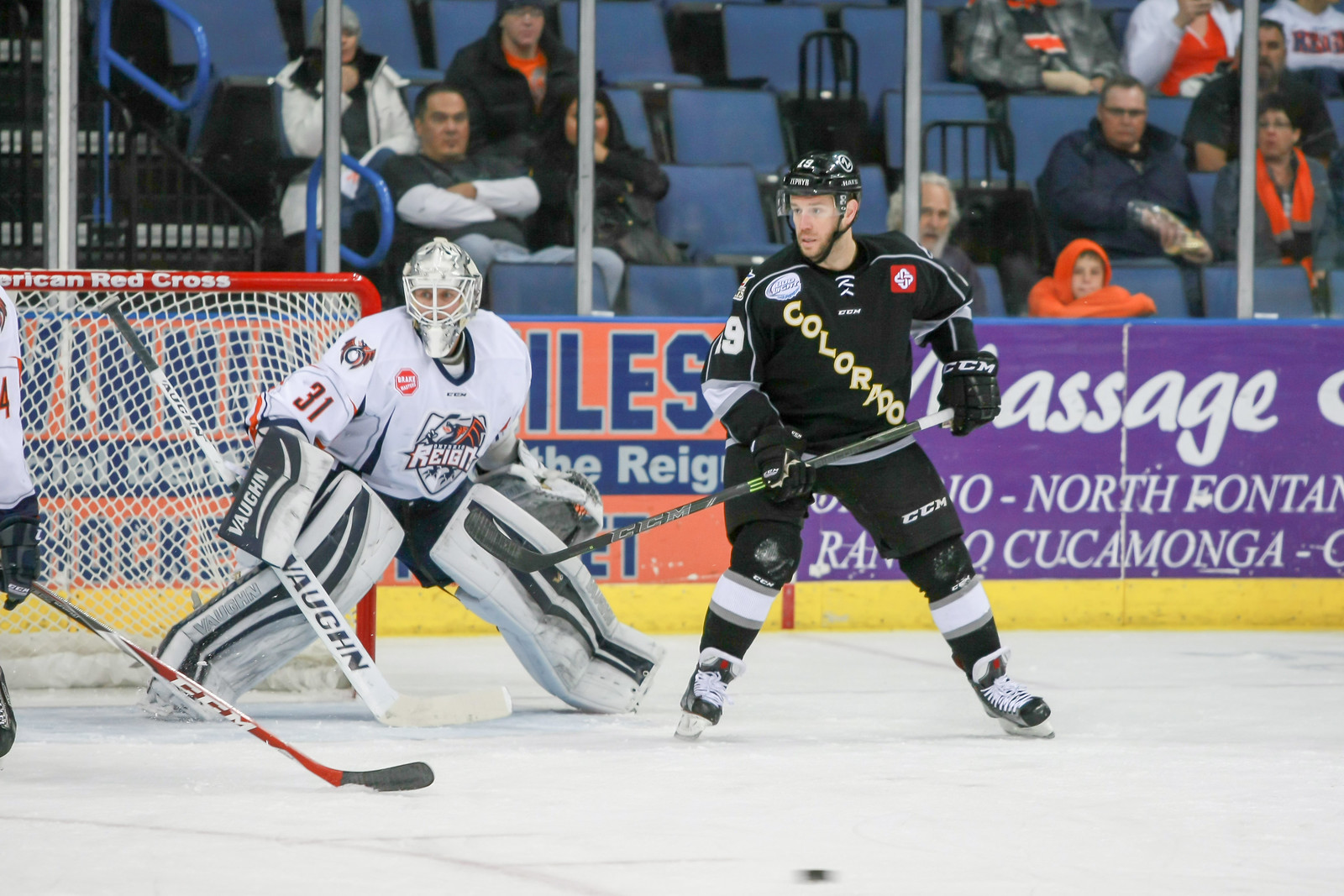In this detailed action shot of a hockey game, we have a vibrant scene unfolding on the ice. Central to the image are two prominently visible players: one in a full black uniform accented with yellow, bearing the word "Colorado" down the front, equipped with shoulder pads and a face mask; and another player, the goalie, dressed entirely in white, from his helmet to his jersey, which features the logo of a dragon and the word "Ontario." The goalie stands with legs apart, eyes intently focused downwards where the puck is visible near the bottom right of the frame. Partial glimpses of another player are present, showing just a glove and hockey stick on the ice.

In the background, there are stands filled with spectators behind a glass partition, although the crowd's subdued demeanor suggests either the game has just begun or the excitement is currently low. Blue chairs in the stands can be seen. Surrounding the rink, various sponsor banners are displayed, though only a massage sponsor's banner is legible among them. The scene captures a moment rich with tension and anticipation as the game is in motion.